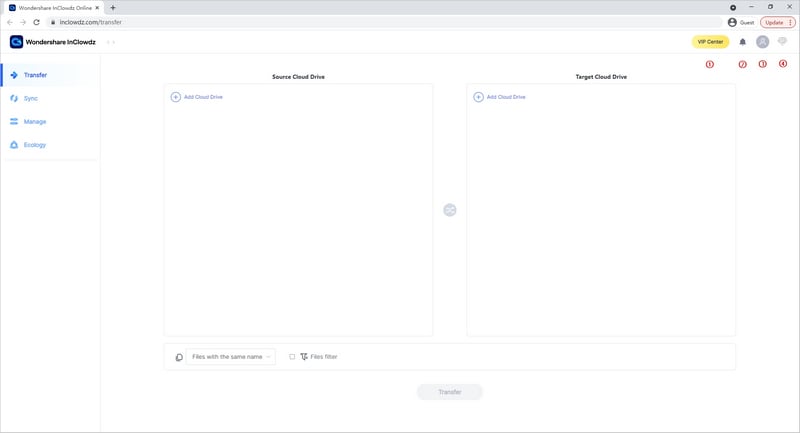The image depicts an interface designed for managing cloud storage and transferring files. A prominent grey navigation bar spans the top of the interface. Beneath it, a large grey search bar displays the text "inclouds.com-transfer," with an "Update" button inside a long red oval shape positioned to the right of the search bar. Below this section is a blue square labeled "Wondershare Clouds" and a nearby yellow circle. 

On the left side of the interface, beginning from the top, a vertical menu features the word "Transfer" highlighted with a blue background. Below it, the menu items "Sync," "Manage," and "Ecology" are listed. Adjacent to this menu, on the right, is a section labeled "Source Cloud Drive" in small black text. This area includes an empty box with an option to "Add Cloud Drive." On the far right, another section is labeled "Target Cloud Drive" in black text. Below this, a larger square provides another option to "Add Cloud Drive."

At the bottom of the interface, there is a light grey circular button with the word "Transfer" inside it.